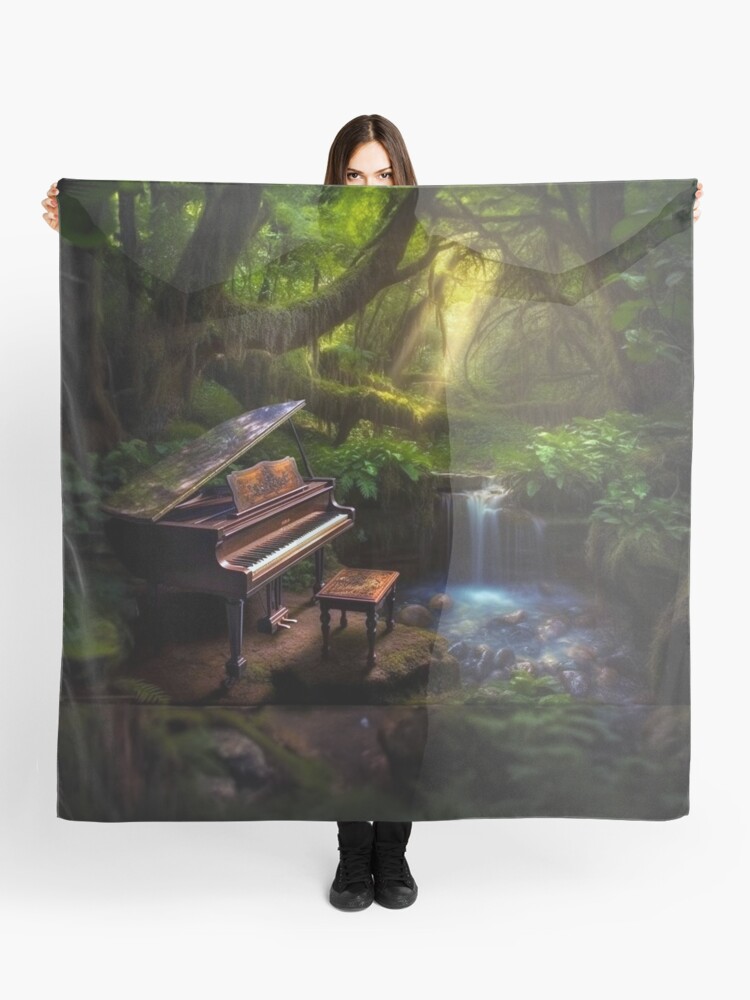A woman stands in front of a solid white-gray background, holding up a semi-transparent cloth or drape. Her silhouette, including the outline of her arms, body, eyes, and feet, is faintly visible through the cloth. The entire surface of the cloth features an enchanting, dreamlike design of a dark, fantasy green forest, adorned with trees and swinging vines. In the midst of this mystical setting, a brown classical piano sits near a gently flowing creek and a soft waterfall, evoking a fairy-tale ambiance.